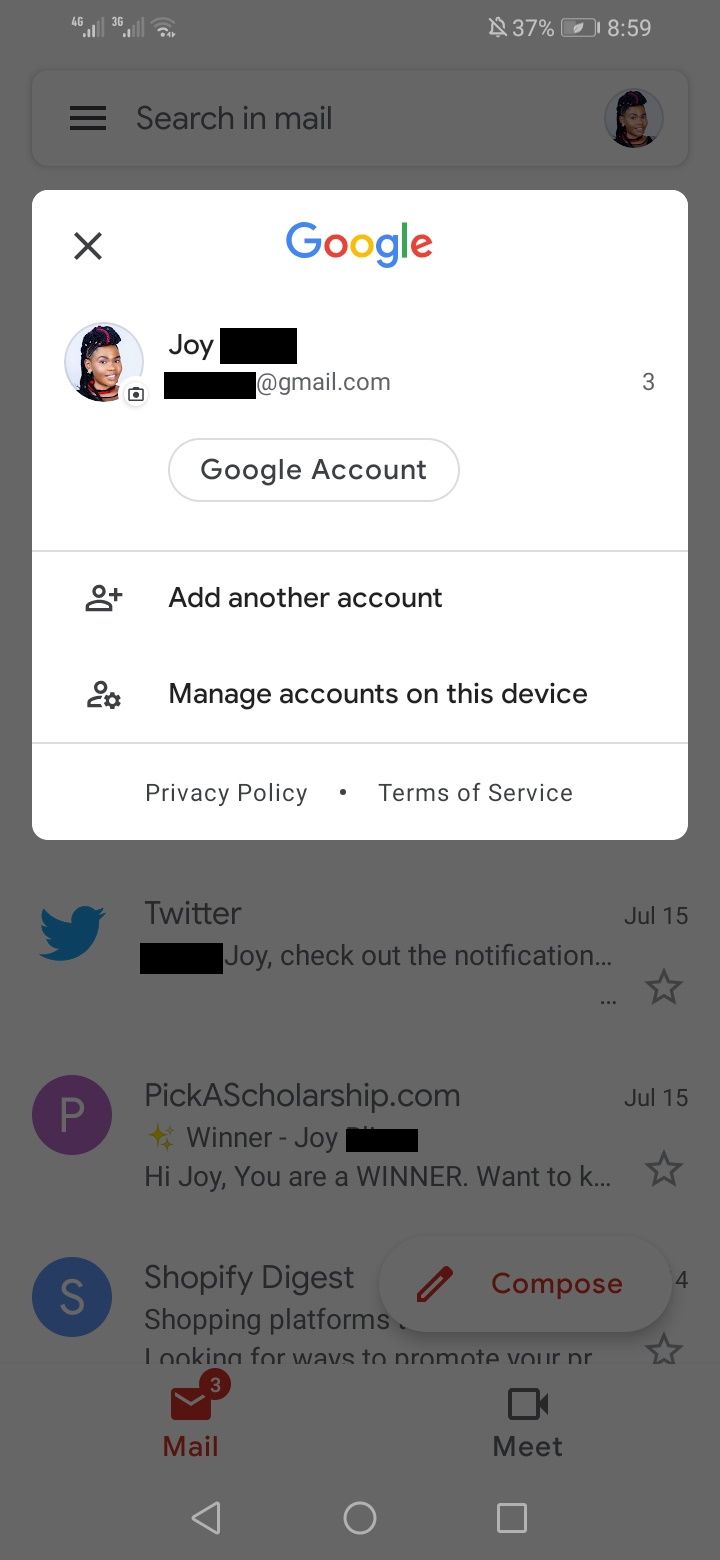The image depicts a smartphone screen belonging to a user named Joy, who is currently accessing their Gmail account. At the top of the screen, various indicators display a weak Wi-Fi signal, a faint mobile data signal, a battery level at 37%, and a phone set to silent mode. The current time is 8:59.

Joy's Gmail interface is open to the "Manage Your Google Account" section, showing a partially obscured profile picture of a black woman, identified as Joy, with her surname and email address redacted to maintain privacy. Below, Joy has three new, unopened emails, prominently listed. The emails include a notification from Twitter sent on July 15th, a congratulatory message from BiggerScholarship.com, and a promotional email from Shopify Digest.

In the background of the Gmail interface, Joy's profile image reappears accompanied by the search email bar, reaffirming this as her personal account portal.